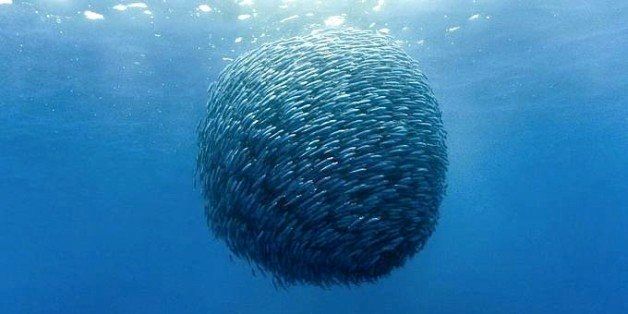This horizontally aligned rectangular image captures an underwater scene in the middle of the ocean with a pristine medium blue background. At the top of the picture, where the water's edge is visible, there are splashes and bubbles showing white, possibly from birds or the interaction with the surface. In the center of the image is a large, spherical formation that appears textured and fuzzy towards the bottom. This formation is a school of countless tiny silver and bluish-silver fish, swimming in unison in a circular, almost spherical manner. The light filtering through the water from above reflects off the fish, creating a shimmering effect, particularly towards the top of the circle. The overall impression gives a sense of movement and the natural beauty of underwater marine life.